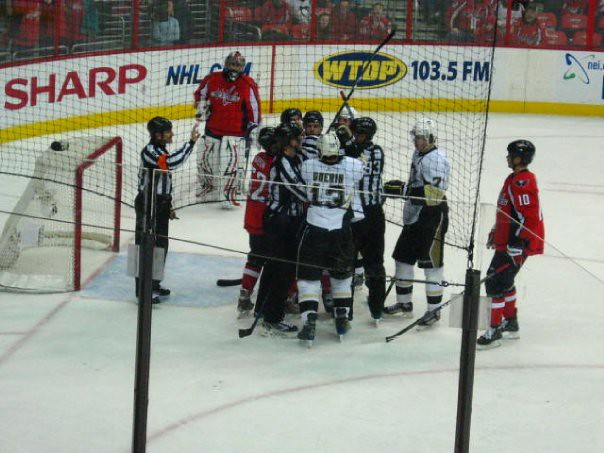The photograph captures a high-intensity moment during an indoor ice hockey game. In the center, a group of players from two opposing teams stands near the net, possibly engaged in a heated exchange or a fight. The players and officials are clearly differentiated by their uniforms. One team is dressed in white jerseys with black trousers, white socks, and white helmets, while the other team is in red jerseys, black trousers, red socks, and black helmets. The officials, identifiable by their black and white vertically striped shirts and black trousers, along with black helmets, try to manage the situation.

The ice rink is well-defined, with white ice accented by a red stripe. Two metal poles in the foreground appear to support a mesh net that protects spectators. Behind the action, a low rink wall painted white with a yellow border is lined with various advertisements. Prominently, "SHARP" appears in bold red letters, followed by "NHL" in blue italics, and further along, a dark blue oval with "WTOP" in yellow capital letters. Adjacent to it, "103.5 FM" is displayed in blue. The top of the photograph reveals the front row of stadium seating, where fans are either seated or standing, with the rest of the stands cut off from view.

Overall, the image vividly portrays a tense and dynamic scene amid the organized chaos of an ice hockey game, framed by the rink's commercial surroundings and the engaged spectators.